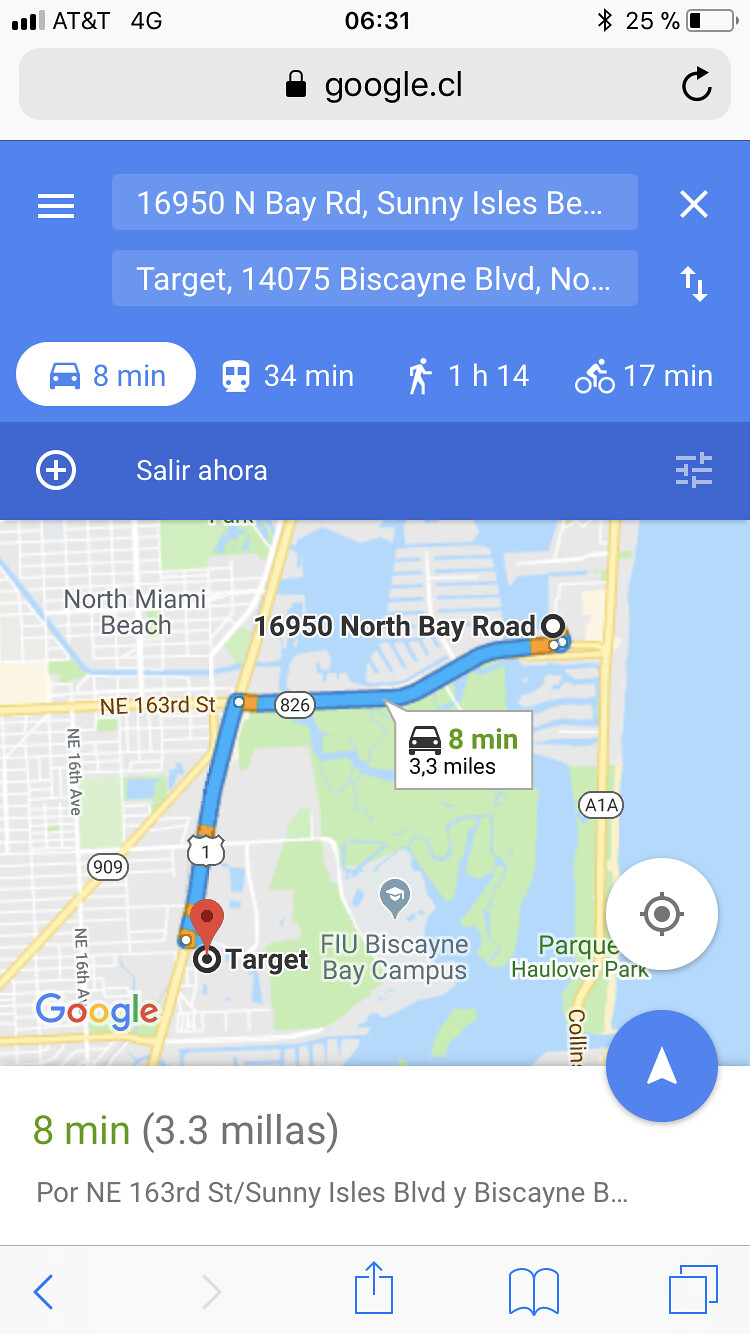This image is a screenshot from a smartphone displaying a Google Maps route between 16,950 North Bay Road, Sunny Isles, and the Target store located at 16,075 Biscayne Boulevard. The map offers various travel options: 34 minutes by bus, 1 hour and 14 minutes on foot, 17 minutes by bicycle, and 8 minutes by car. A blue line illustrates the route, predominantly following Route 826 and U.S. Route 1. The right side of the map shows the ocean, while the travel details—distance of 3.3 miles, travel time, and the Google logo—are located at the bottom. Additionally, the status bar of the screenshot indicates the service provider as AT&T, the current time as 6:31, and the battery level at 25%.